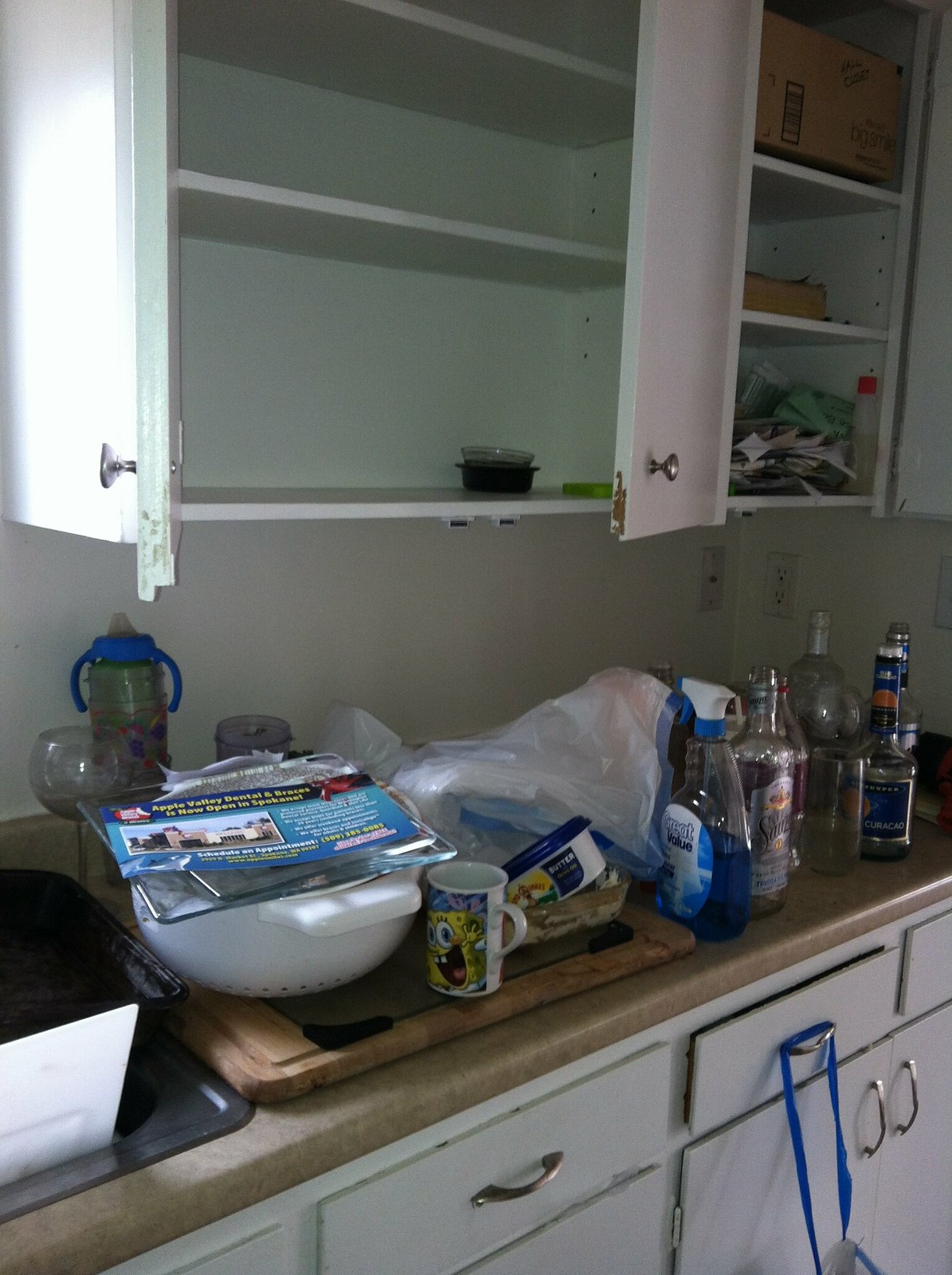The image depicts a well-used kitchen space with various items scattered around. At the top of the scene, there is a white cabinet with three shelves. The top two shelves are empty, while the third shelf houses a black container with a green lid situated at the back. To the right of this cabinet, there are additional white shelves. The top shelf holds a large brown box, the middle shelf contains a medium-sized brown box, and the bottom right shelf is cluttered with paper scraps.

In the center of the image is a brown countertop. On this countertop rests a bottle of Great Value cleaning spray, a SpongeBob-themed cup, a pasta strainer, and several alcohol bottles clustered on the right side. The left side of the countertop is home to a sink, above which a white trash bag with blue lining is visible. Below the sink and countertop, several closed drawers are present, one of which has a blue-strapped trash bag hanging from it. Finally, a few water bottles are situated towards the back left of the scene, resting against the white wall.